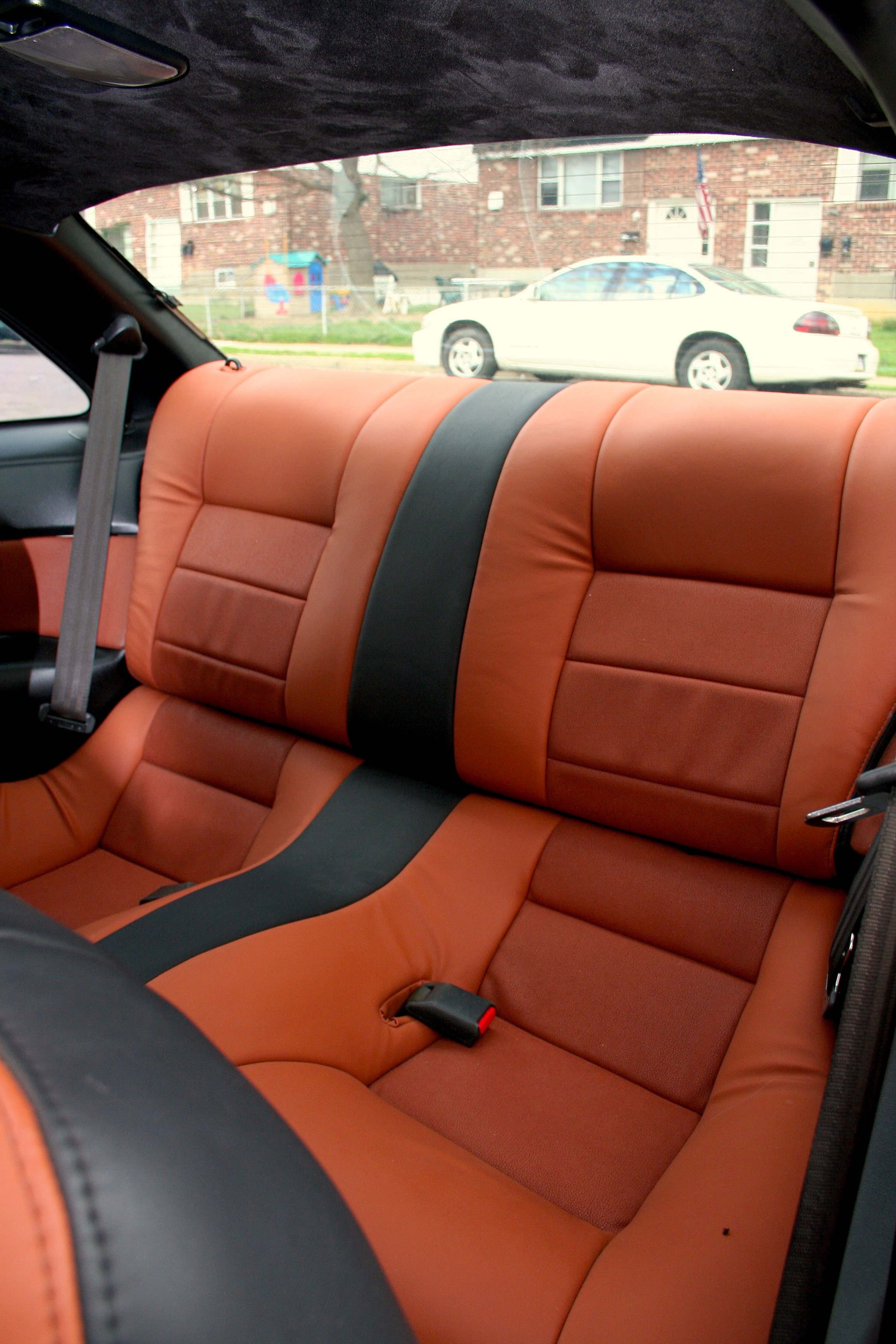This vertically aligned rectangular photo captures the interior of a vehicle from just in front of the driver's seat. The focus is on the backseat area, featuring two rust-colored leather bucket seats separated by a black strip of leather. These seats look very comfortable, dipping down in the center where one would sit, and have gray seat belts visible on either side.

In the lower left-hand corner of the image, the curve of the top of the driver's seat is noticeable, with a distinctive orange front and a black top. The vehicle's roof appears to be made of a black, possibly satiny material. 

Through the rear windshield, a white sedan is parked across the street. Beyond the car, a chain link fence lines the sidewalk, with grass and red brick apartment buildings in the background. These buildings have white doors and windows, with some displaying a flag and housing children's playhouse-style toys with green roofs and brown sides. The partially shown seatbelt metal part and a bit of the side back door, which is black with an orange stripe, add to the detailed interior view.